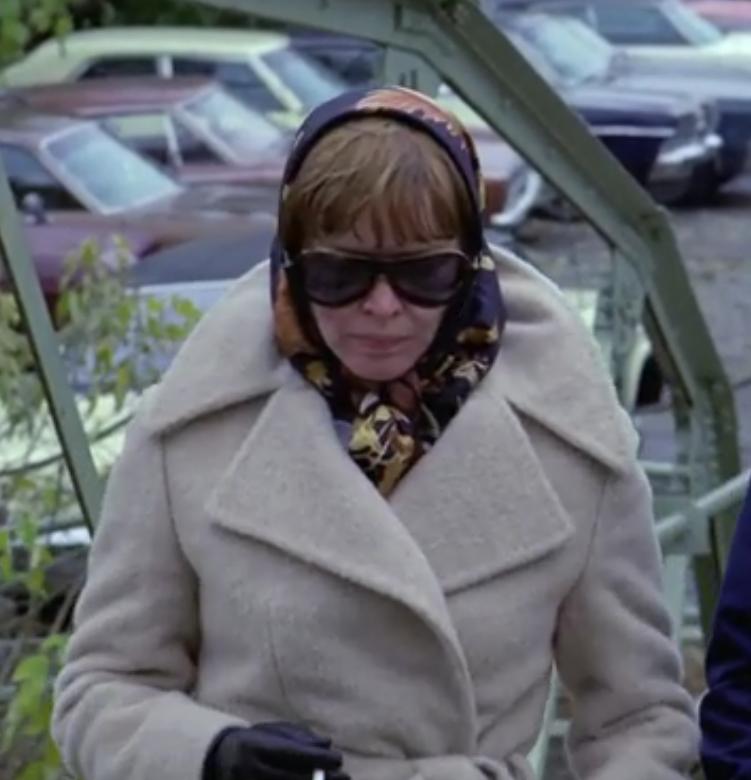In the center of this daytime outdoor image, a woman stands in a parking lot on an asphalt road. She's dressed warmly in a thick beige, winter coat and a dark-colored scarf that wraps around her head and is tucked into her collar. The woman is also wearing large, round-edged sunglasses and black gloves. One hand holds a cigarette. Her lips are tightly pressed together as she looks down slightly. Behind her, several cars are parked, and trees are visible. The colors in the image include tan, gold, black, brown, green, maroon, red, and gray. There is no text present in the photograph.